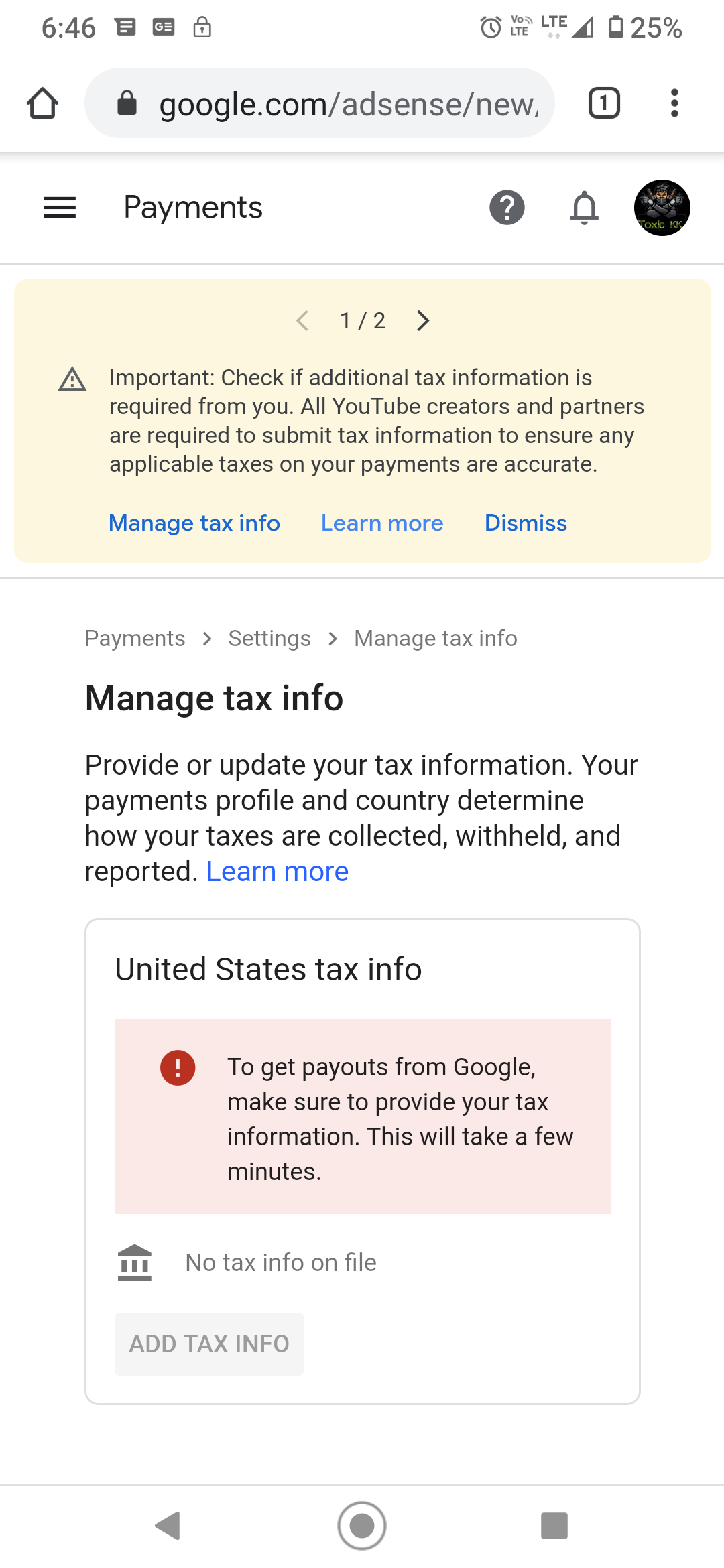The vertical rectangular image, likely captured from a phone, depicts a webpage from Google AdSense. At the top of the page, within the search box, is the partially visible URL: "google.com/AdSense/new." The left side of the top section features the word "Payments" in black font.

Beneath this, a horizontal pale yellow box displays the text "1/2" surrounded by greater-than and less-than signs. Adjacent to this, a yellow triangle with an exclamation mark inside serves as a warning symbol. The accompanying black font message reads, "Important: Check if additional tax information is required from you. All YouTube creators and partners are required to submit tax information to ensure any applicable taxes on your payments are accurate."

Below this, in turquoise font, the text "Manage tax info" is clickable. Nearby, the options "Learn more" and "Dismiss" are available, with "Learn more" positioned centrally and "Dismiss" to the right.

Further down, in gray font, the path "Payments > Settings > Manage tax info" is followed by the prominently displayed black text, "Manage Tax Info." A slightly smaller black font advises, "Provide or update your tax information. Your payments profile and country determine how your taxes are collected, withheld, and reported." This section also includes a turquoise "Learn more" link.

The image also contains another vertical rectangular section labeled "United States Tax Info" in black font. Inside this section, a light pink horizontal box features a red circle with a white exclamation point. The black text inside this box states, "To get payouts from Google, make sure to provide your tax information. This will take a few minutes." Below, in gray font, it states, "No tax info on file," followed by a prompt to "Add tax info."